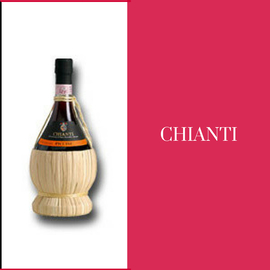The image features a bottle of Chianti wine placed prominently on the left side against a white background. The bottle itself is black with a beige-colored wrapping around its bottom, along with an orange portion on its label and a black cap. It appears to be held in a traditional straw basket specifically shaped to fit the bottle. The right half of the image contrasts sharply with a red background displaying the word 'Chianti' in bold white letters, centered in the middle. A hard, dark drop shadow behind the bottle adds depth to the visual composition, making the advertisement vibrant and eye-catching.